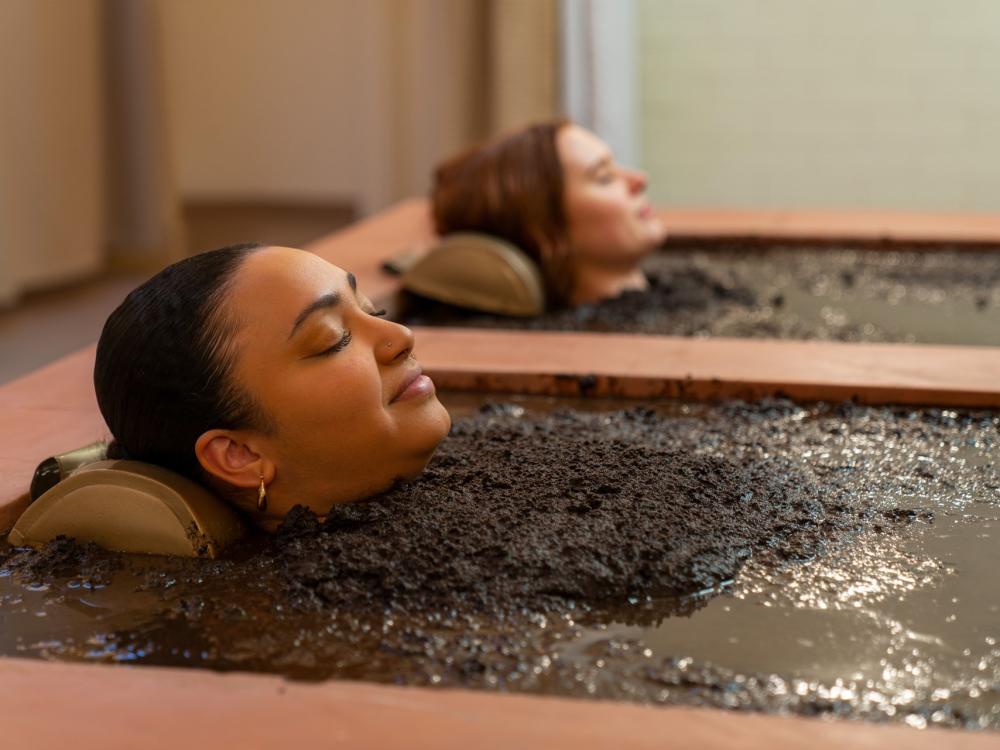In this indoor spa scene, the photograph captures two women submerged in a luxurious, rich dark brown mud bath, each in their own wooden tub, appearing relaxed and serene with their eyes closed and slight smiles on their faces. Their heads rest comfortably on brown cushions. The woman in the foreground, who wears gold hoop earrings, is clearly featured, while the second woman is slightly blurred in the background. Both women are submerged up to their necks in the thick mud, which envelops them fully, creating an impression of indulgent relaxation. The setting is bright but blurred, focusing the viewer’s attention on the tranquility and detailed expressions of the women in their soothing spa experience.